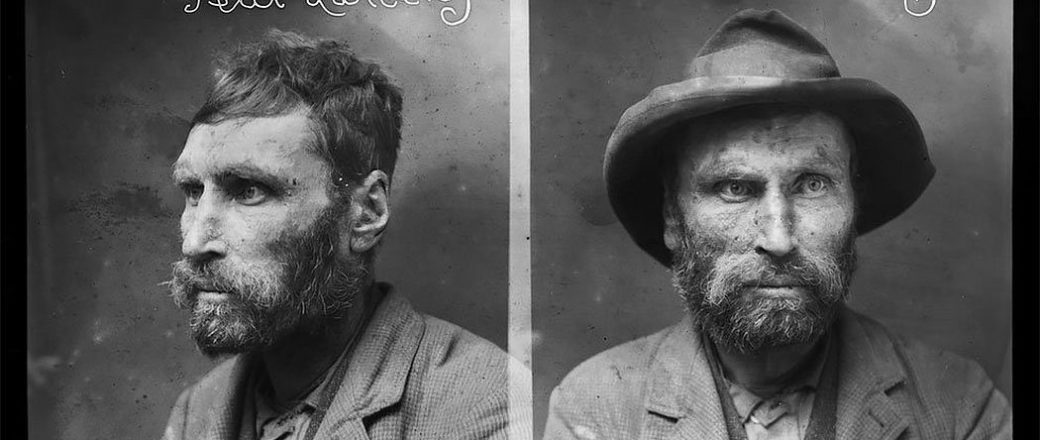This striking black-and-white image showcases two side-by-side photographs of the same man, evoking a sense of historical mystique reminiscent of the late 1800s to early 1920s. In both photographs, the man presents a serious, almost grim expression, with a neatly trimmed beard and mustache. 

In the left-hand photograph, the man, who bears a resemblance to Vincent van Gogh or an old-time cowboy or farmer, stands with his head slightly turned to the camera's left. He dons a collared jacket and shirt, showcasing a somewhat unkempt appearance with short hair. His face appears weathered, possibly indicative of skin issues, adding to the rugged and timeless quality of the image.

In contrast, the right-hand photograph features the same man wearing a hat, synonymous with the era's frontier exploration. In this image, he faces straight ahead, though his eyes divert slightly to his left, maintaining the serious demeanor seen in both images. The background is uniformly dark and non-descript, allowing the viewer to focus entirely on the man's stoic presence, uninterrupted by any text or other distractions. This compelling dual portrait captures the essence of a bygone era, immortalizing the man's enduring and stern visage.